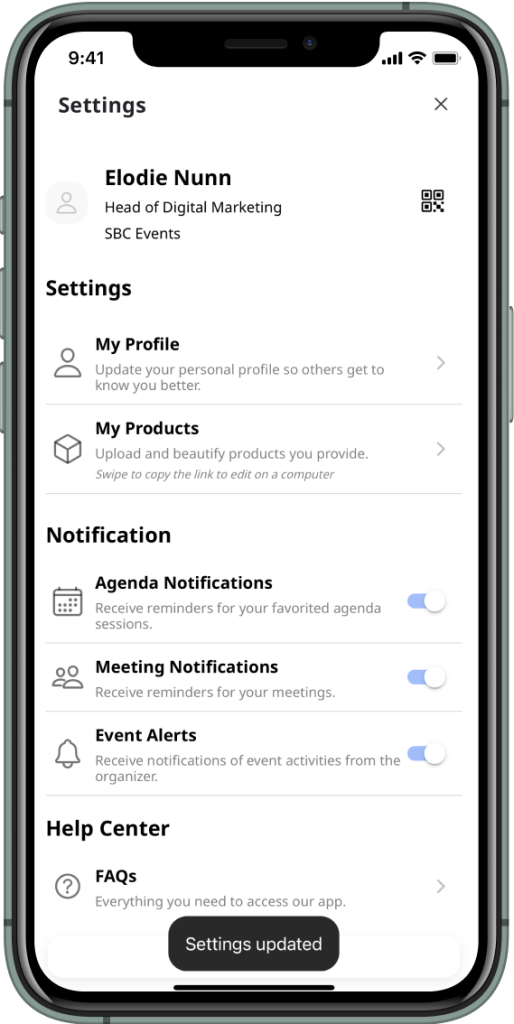A screenshot of an app's settings section. At the top left, the heading "Settings" is displayed, while a dark grey "X" icon is positioned at the top right corner. Below, the name "Lodi Nunn, Head of Digital Marketing, SBC Events" is featured, followed by another "Settings" heading. The section is divided into several categories:

1. **My Profile**: Prompts users to update their personal profile so others can get to know them better.
2. **My Products**: Allows users to upload and enhance the products they provide.
3. **Notifications**:
   - **Agenda Notifications**: Users can receive reminders for their favorited agenda sessions.
   - **Meeting Notifications**: Users can receive reminders for their meetings.
   - **Event Alerts**: Users are notified of event activities by the organizer.

At the bottom, there is a "Help Center" section available for further assistance.